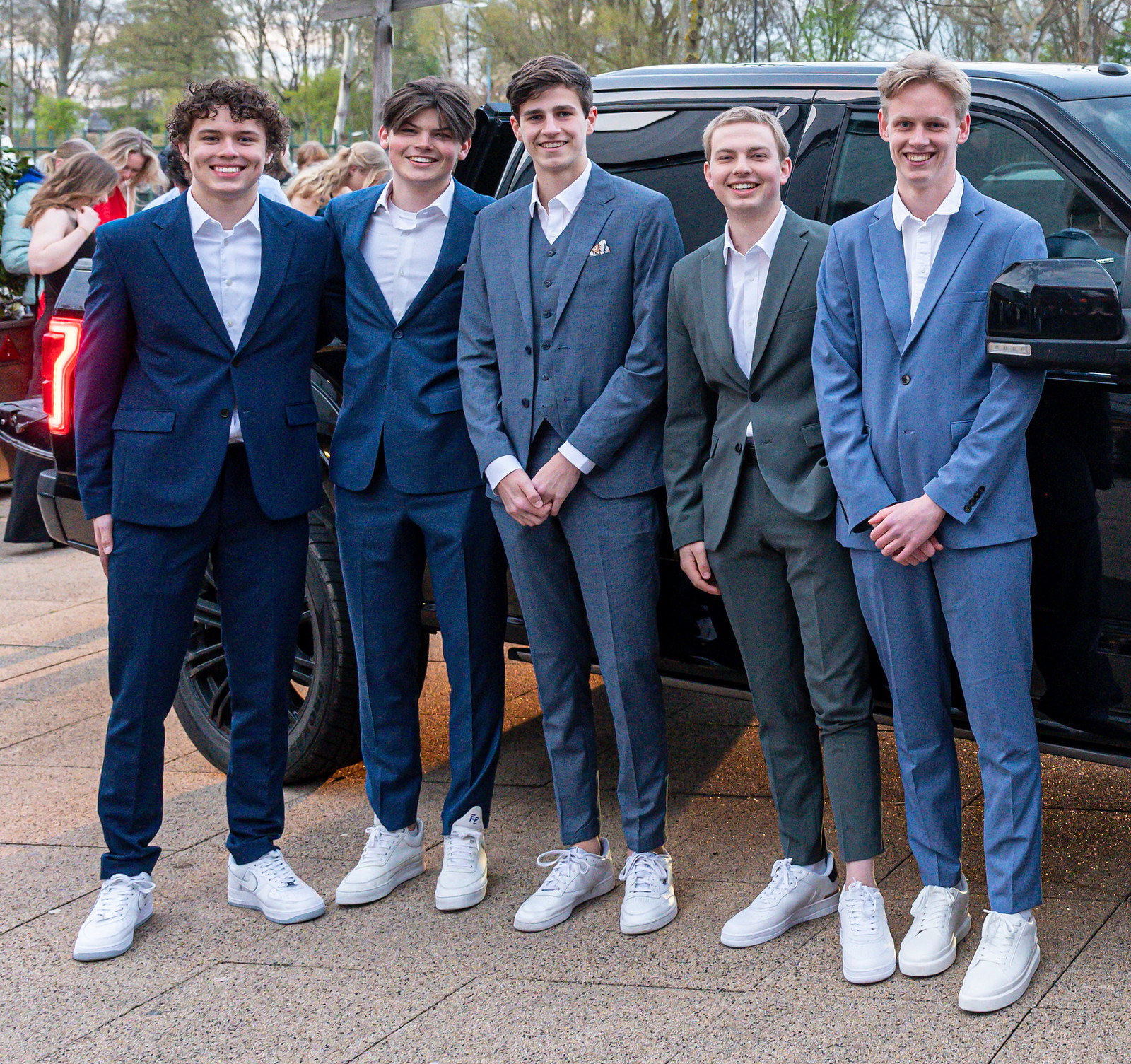This photograph features five young Caucasian men, likely in their late teens to early twenties, standing on a driveway paved with large square tiles. They are all dressed in blue suits of varying shades, with one suit tending towards gray. Each is wearing a white button-down shirt and white tennis shoes, with their ankles visible, suggesting they are either wearing no socks or low socks. The suits are buttoned at the top, except for the boy in the middle who is also wearing a vest and a pocket square, and has his coat unbuttoned. Three of the men have brown hair and two have blonde hair. They are positioned in front of a black SUV with black wheels. In the left background, several women, perhaps mothers, some in long dresses and jackets, are gathered, possibly preparing to take photos. The scene suggests they might be ready for a significant event like a high school prom or dance.